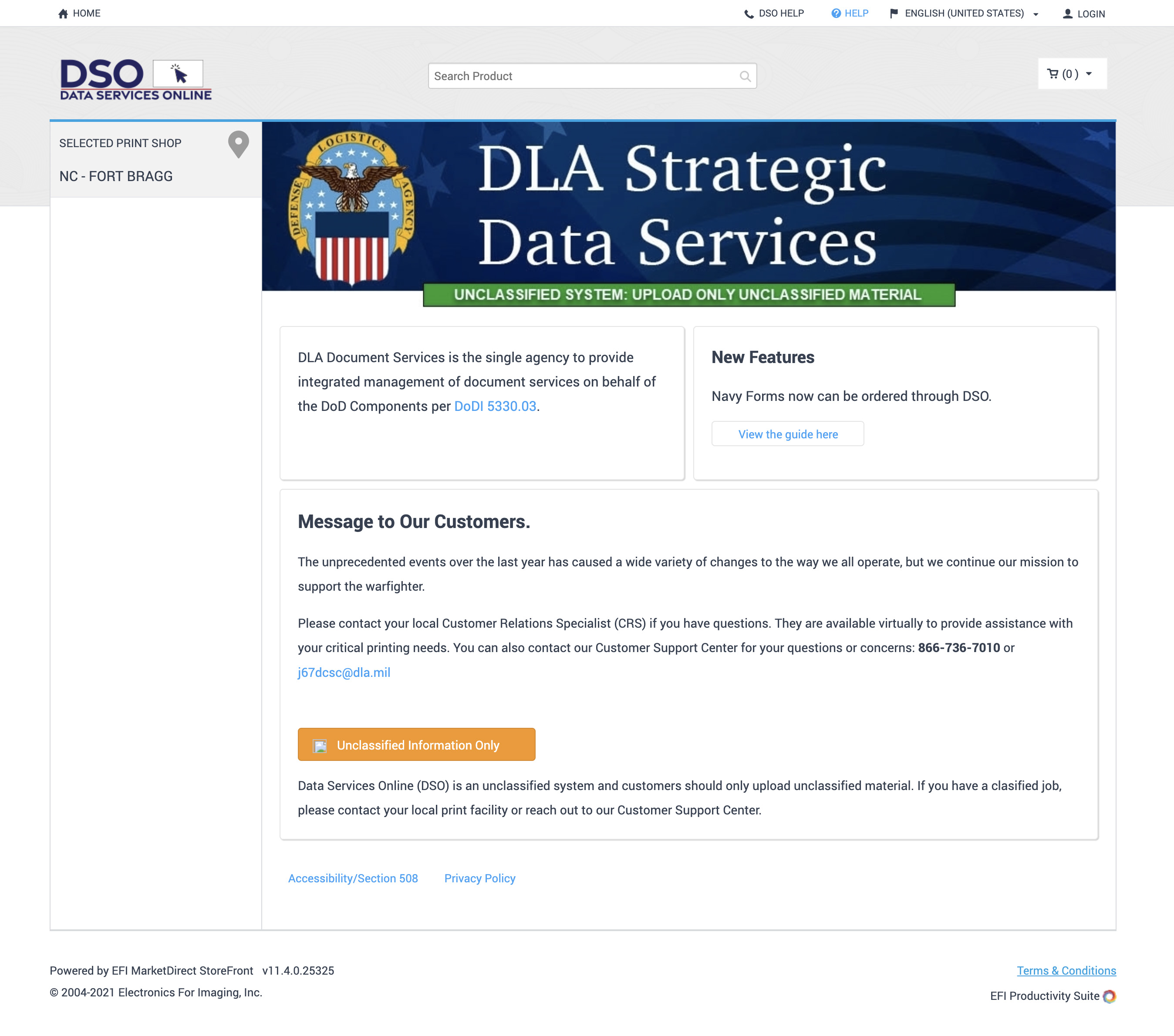Screenshot of the Data Services Online (DSO) Website for Managing Unclassified Data

The image depicts a screenshot of the Data Services Online (DSO) website, designed for managing unclassified data, presumably for U.S. government or military services. The top left corner features the site's logo with "DSO" in prominent blue text, and "Data Services Online" written below it in a smaller font.

At the top center of the page, there's a white search bar for navigating the website. In the top right corner, a shopping cart icon within a white box suggests that users can make purchases or transactions. The main page is set against a white background and is dominated by a large blue box located at the top center. This box showcases an American flag as the background and displays "DLA Strategic Data Services" in large white text at the center. To the left of this text is a logo comprising an American flag, an eagle, and a blue banner with white stars, representing the service.

Below the blue box, a small green box contains the text "Unclassified System. Upload only unclassified material" in white, emphasizing the nature of the data permitted on the site. The remainder of the page provides detailed information on how to upload data and outlines the features and functionalities of the website. Additionally, a message offers contact information for customer support.

At the bottom center of the page, a large orange box with white text reiterates the site's unclassified nature with the message, "Unclassified Information Only," reminding users to upload only unclassified materials.